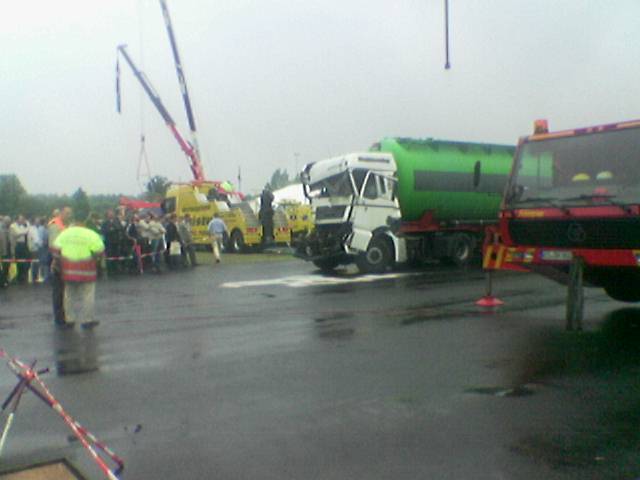The photograph, taken on a rainy and somewhat foggy day, captures a scene of an industrial or construction area following a vehicular accident. The sky is overcast and white, with water pooling on the black asphalt ground. To the left, a crowd of people, including workers, stands behind a small barrier, observing the aftermath. In the center, a large white truck with a green tanker has sustained significant front-end damage; its door hangs off and the front window is severely smashed. On the right side, a bright yellow tow truck equipped with a crane stands close to the wreck, with a man walking toward it from the crowd. Further to the right are a semi-truck with a green transport bed and a red emergency vehicle. Emergency crews are actively managing the situation, adding a sense of urgency and response to the chaotic scene.